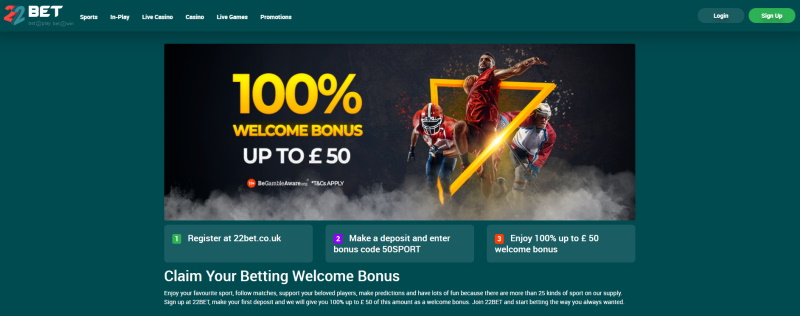**Caption:** "The homepage of 22bet features a striking teal-green background, prominently highlighting its sports betting and online casino services. At the top, users can navigate through various sections including Sports, In-Play, Live Casino, Casino, Live Games, Promotions, with options to Log In or Sign Up positioned on the right. The central banner showcases dynamic, generic athletes: an American football player, a basketball player in mid-dunk, and a hockey player. Beneath this image, a promotional message offers a 100% welcome bonus up to £50. The instructions read: 'Register at 22bet, make a deposit, and enter your bonus code 50SPORT (5-0-S-P-O-R-T). Claim your 100% welcome bonus up to £50.' Additional legal details follow, indicating that 22bet is a UK-based sportsbook."